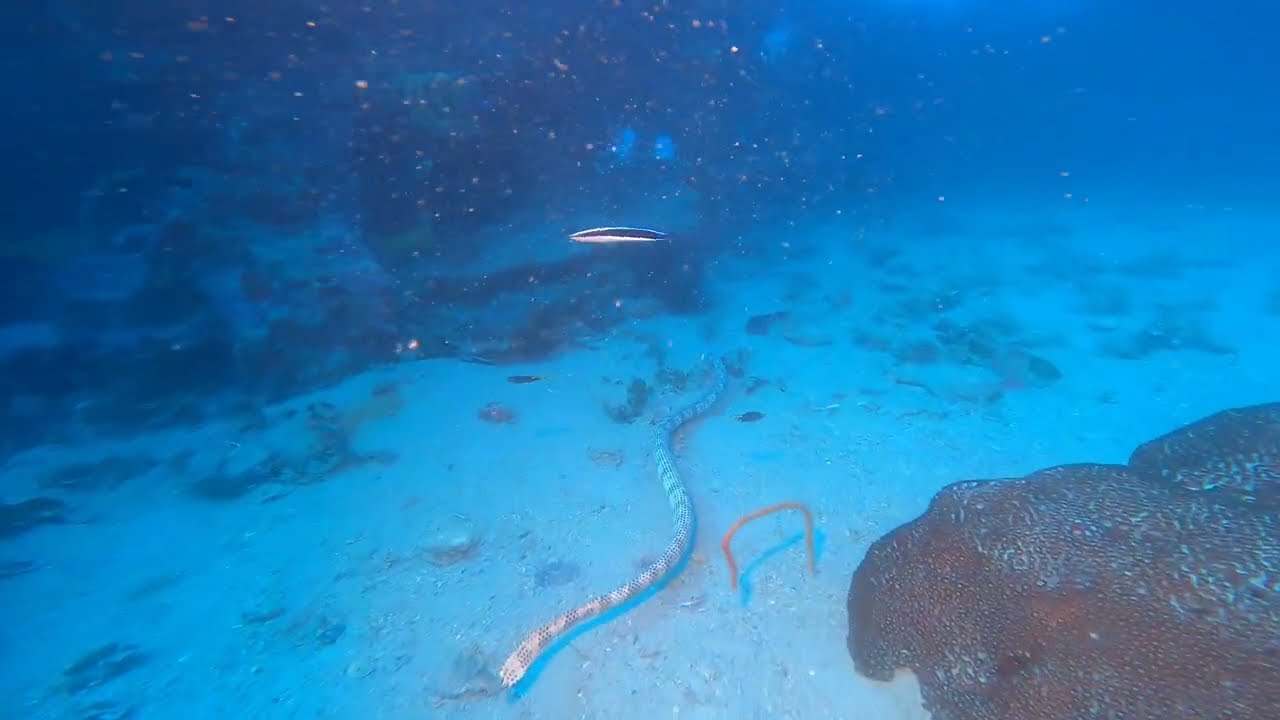This underwater photograph captures a serene ocean floor scene dominated by a few key elements. At the center, a striking black-and-white striped sea snake or eel winds its way across the sandy, rock-strewn seabed, its distinctive pattern drawing immediate attention. Accompanying this creature is a black-and-white striped fish, adding to the visual interest with its similar color palette. 

In the foreground and scattered throughout, smaller rocks and debris dot the sandy bottom, providing texture and complexity. The background features a large rock formation or possibly coral to the left, contrasting with the darker, deeper blue waters to the top right. The water itself is slightly murky, filled with particulate matter that reflects the soft, filtered light penetrating from above.

Adding to the mystique, there's an indistinct object that resembles either a metal structure or another sea creature looping into the seabed, forming a U-shape. Despite the blurriness typical of underwater photography and the lack of identifying information about the location or the photographer, the image gracefully captures the quiet complexity of marine life.